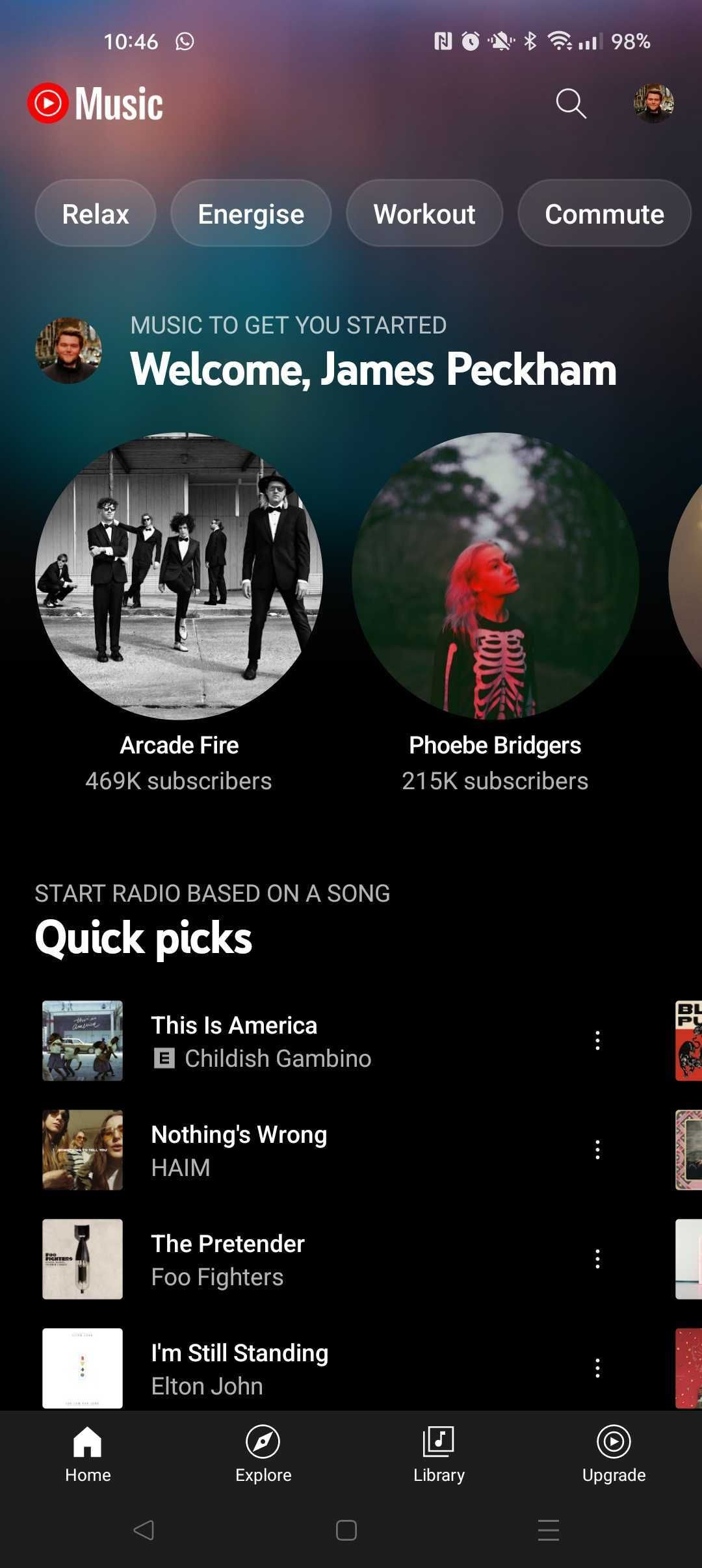A detailed smartphone screenshot captures various elements of a music app at 10:46, with 98% battery life and active Bluetooth and alarm clock icons at the top. The screen title "Music" is prominently displayed in white letters. Categories available for exploration include "Relax," "Energize," "Workout," "Commune," and "Music to Get You Started." The welcome message reads, "Welcome, James Peckham."

A circular black and white photo featuring numerous people represents the band Arcade Fire, noted to have 469,000 subscribers. Below this, another image showcases a white woman with blonde hair wearing a top decorated to resemble a skeleton's rib cage, identified as Phoebe Bridgers with 215,000 subscribers.

Options to "Start radio based on a song" and "Quick Picks" are listed with specific tracks:
- "This is America" by Childish Gambino
- "Nothing's Wrong" by HAIM (all letters capitalized)
- "The Pretender" by Foo Fighters
- "I'm Still Standing" by Elton John

Navigation options "Home," "Explore," "Library," and "Upgrade" are positioned at the bottom of the screen. Some cover art sections are partially visible on the right side but are cut off from the viewer's sight.